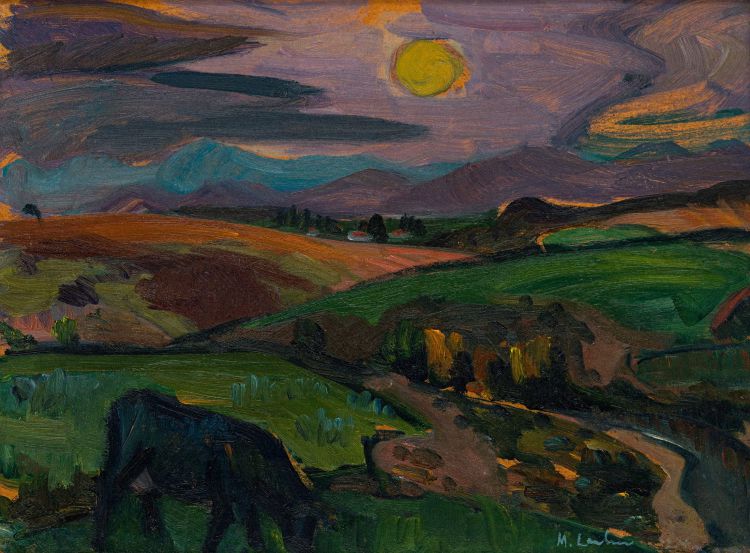The painting is a vibrant and colorful impasto depiction of a hilly landscape, exuding a somewhat childlike yet highly sophisticated charm. Starting from the top, the sky bursts with an array of colors, including light and dark blues, purples, grays, and swirls of orange and green. A striking yellow sun sits at the top center, with hints of green and orange brush marks giving it a swirling appearance. Below the sky, a mountain range colored in shades of plum and purple stretches across the scene, with touches of turquoise blue just above, perhaps indicating a distant haze or atmospheric effect. 

Descending into the landscape, we find rolling hills painted in varying hues. The upper portions of some hills are tinged with brown, suggesting dirt, while the lower regions shift into lush greens representing grass. Interspersed throughout are swathes of orange and brown, adding a rich texture to the fields. Vertical blue stripes on some hills denote grassy areas. At the bottom left of the painting, a black four-legged animal, likely a cow, grazes peacefully. 

Additionally, there is a strip of grayish color resembling a river that meanders between the front hillsides, adding depth and movement to the scene. The painter's signature, an elegant blue inscription featuring the letters M and L followed by squiggles, is located in the lower right-hand corner. Overall, this detailed painting captures the dynamic beauty of the landscape through its bold use of color and texture.